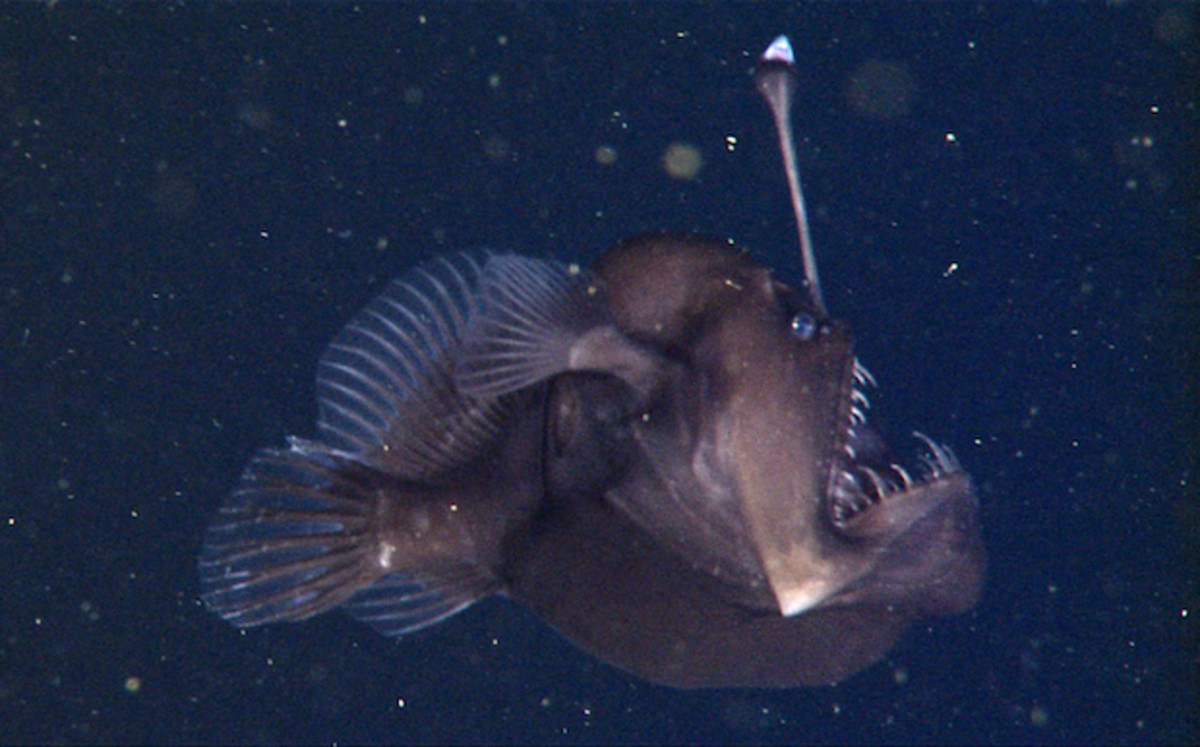This image vividly captures a side view of a monstrous-looking anglerfish submerged in deep ocean water. The fish, predominantly brownish-beige, has a hump-like shape, with a flat, angled base. Its most striking feature is the long, sharp white teeth protruding from its open mouth, resembling fangs. Buggy eyes add to its grotesque appearance. Sticking out from between its eyes is an antenna-like appendage, topped with a bioluminescent, fluorescent blue bob, used to lure prey. The semi-transparent fins are visible, set against a dark, blackish-blue ocean background. Scattered throughout the water are yellow, blue, and green spots and bits of debris, enhancing the eerie atmosphere of the deep sea.